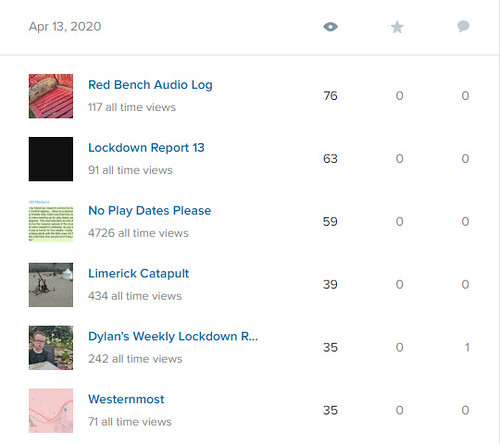At the top of the page dated April 13, 2020, there are several icons: an eye icon, a star, and a comment bubble. Directly below is a list of six reports or titles, each accompanied by an image. The titles are written in blue, and each entry includes detailed view, star, and comment counts.

1. **Red Bench Audio Log**: The accompanying image is of a red bench. This report has been seen by 76 people, with no stars and no comments.
   
2. **Lockdown Report 13**: This entry features a black square and records 63 recent views and 91 all-time views, with no stars or comments.
   
3. **No Play Dates Please**: The image is a green box with lines across it. It has 59 recent views, no stars or comments, and a total of 4,726 all-time views.

4. **Limerick Catapult**: The image seems to represent a beach-like setting, though it is somewhat unclear. It has been seen by 39 people, with no stars or comments, and a total of 434 all-time views.
   
5. **Dylan's Weekly Lockdown**: This features a white man with short dark hair, wearing glasses and a dark shirt. It has 35 recent views, no stars, one comment, and a total of 242 all-time views.
   
6. **Western Most**: The final entry has a predominantly pink image. It has been viewed by 35 people, with no stars or comments, and has 71 all-time views.